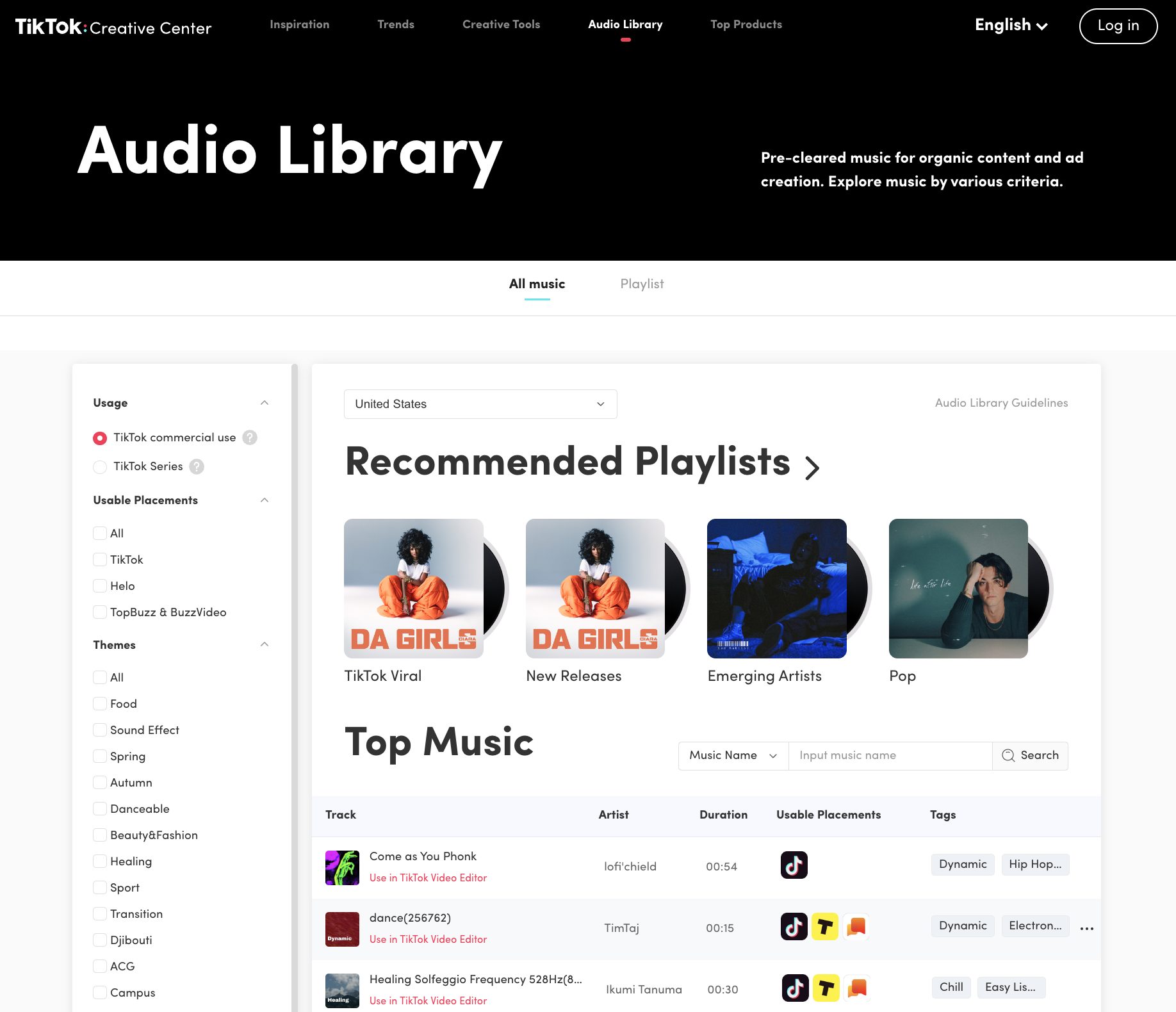The image depicts a minimalist composition featuring a very small box, approximately one inch in height. The box is outlined in dark gray, creating a stark contrast with the primarily white background. Inside the box, the color shifts to light blue, accentuated by a white square situated in the left corner. Below this white square, there's a soft area of green that brings a subtle splash of color. A diagonal white line extends toward the right corner, and the upper right corner of the box appears slightly folded down, giving the impression of the corner of a piece of paper. This simple yet evocative image resembles the placeholder graphic typically used when a photo has been removed or is missing.